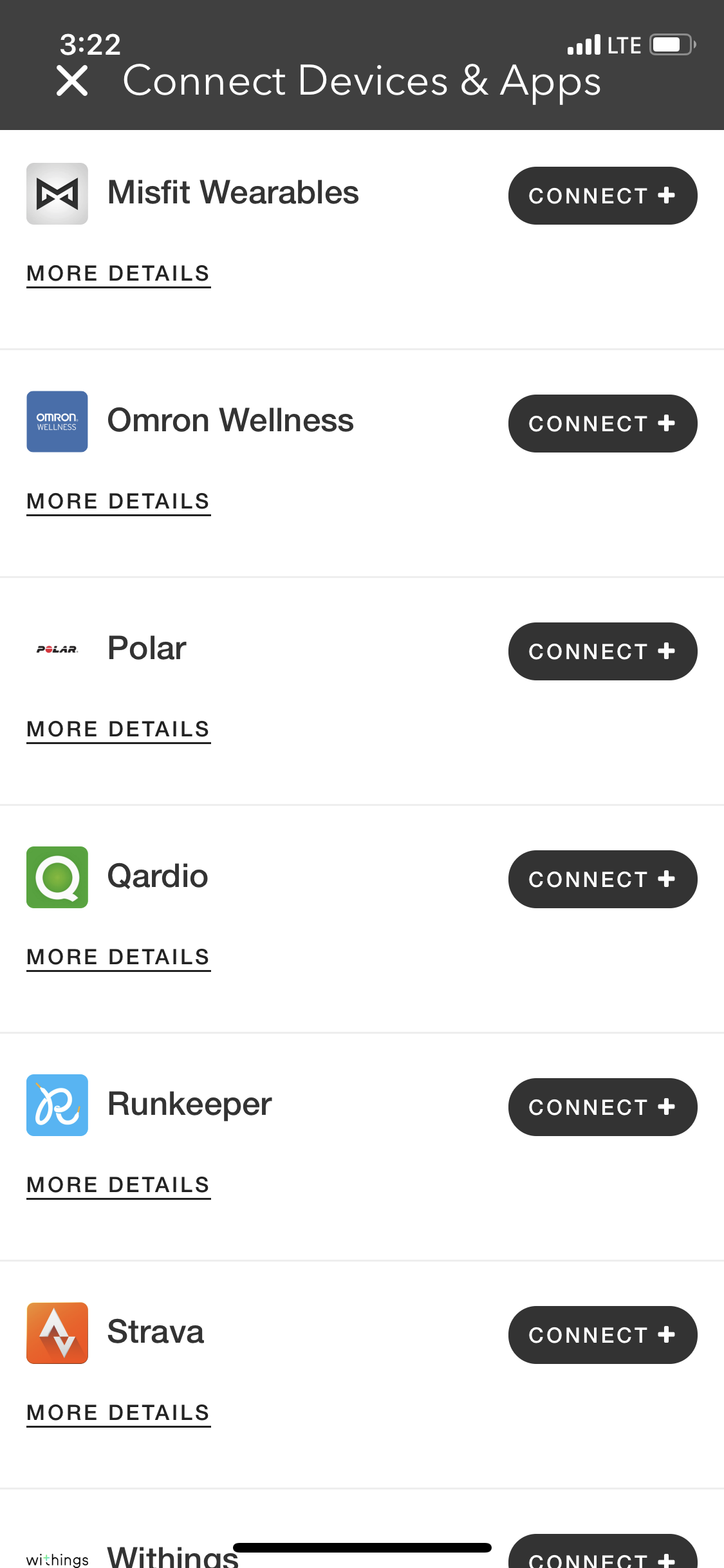In the image, the top portion is a grey section with the number "322" prominently displayed. To the right, there's a grey square followed by the word "Misfit Wearables," indicating a connection to devices and apps. Next, there's a blue square that possibly represents an option to get more details about connecting with this device.

Below, the sequence continues with another grey square displaying the word "Polar," suggesting further fitness tracking connectivity options. A green shadow is associated with the "Connect Cardio" feature. Further along, there is a mention of "Windkeeper," highlighted with a blue square for additional details.

There is a prominent dark oval, possibly an element to draw attention to a specific feature or section. Adjacent to it is an orange section related to "Strava," which includes options to connect and manage wellness tracking.

Wrapping up the visual description, the entire background of the image is a clean white, providing a minimalistic and uncluttered canvas for the various elements displayed.